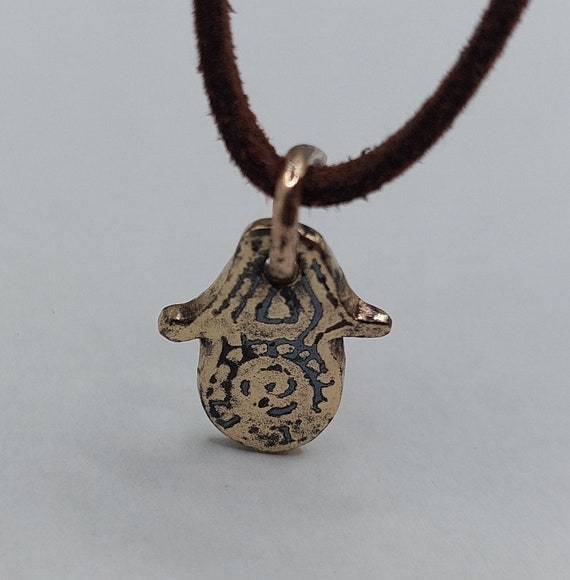This image depicts a close-up of a necklace set against a gray background. The necklace features a fuzzy brown upper strap that appears to be stretchy, almost like a headband. This brown strap seamlessly transitions into a copper chain. Hanging from this chain is a distinct pendant with a gold-tone finish. The pendant is intricately designed, resembling a house or clock shape with a round bottom and a triangular top, akin to a hat. The pendant also features black etchings in a square pattern that appear to be aged and slightly worn, contributing to its vintage look. The combination of the brown strap, copper chain, and gold pendant with black accents creates a visually striking piece of jewelry.